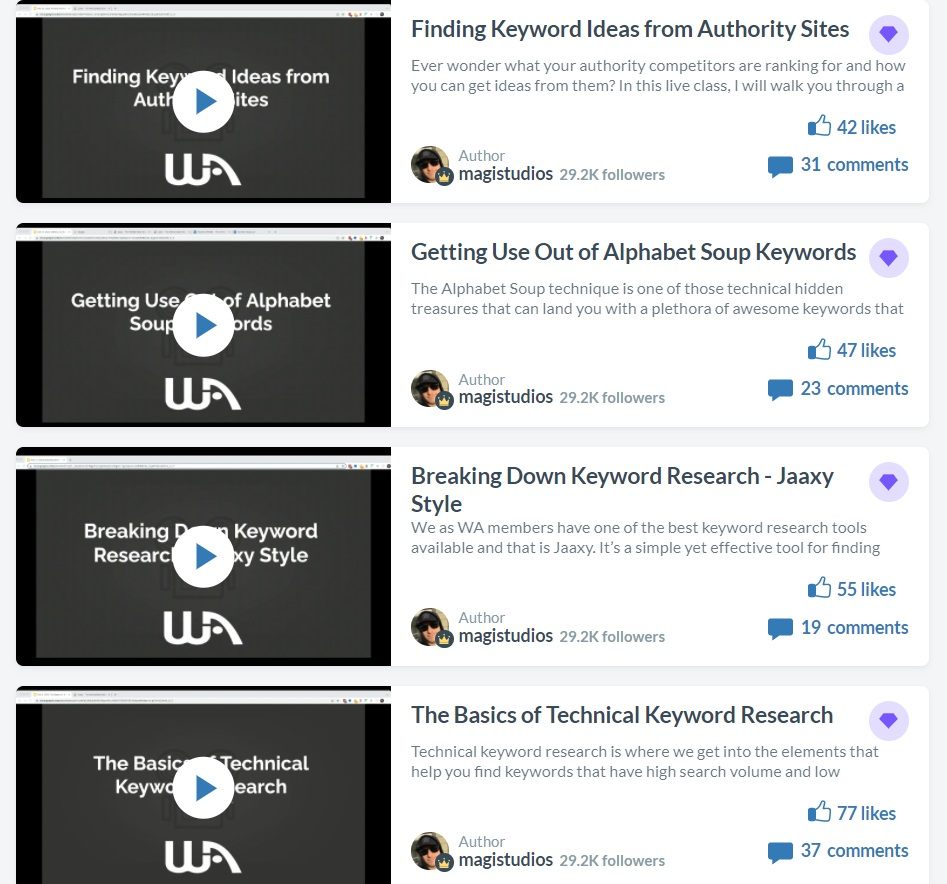The image provides a detailed guide on various methods for conducting keyword research. It features four distinct sections, each accompanied by illustrative black screens with blue arrows set in white circles. 

1. **Finding Keyword Ideas from Authority Sites:** This section offers strategies for identifying high-value keywords by analyzing established authority websites.
   
2. **Utilizing Alphabet Soup Keywords:** Here, the focus is on leveraging the "alphabet soup" method to discover a wide range of keyword variations and ideas.
   
3. **Breaking Down Keyword Research, JAXXY Style:** This part describes the unique approach to keyword research using JAXXY, a specialized tool indicated by the acronym J-A-A-X-Y.

4. **The Basics of Technical Keyword Research:** The final section introduces fundamental concepts of technical keyword research, targeting more advanced SEO techniques.

All these insights are presented by Magic Studios, a reputable entity with 29,000.2 followers, whose posts consistently receive positive feedback from the user community.